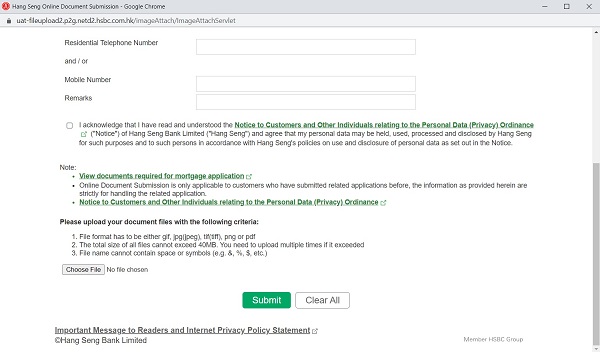In this image of a Google Chrome window, the top left corner displays a red icon resembling a stop sign, adjacent to which are black text characters. In the top right corner of the window, there is a minimize icon, a maximize icon, and a black "X" for closing the window. Below this gray bar, extending horizontally across the top, there is a light gray bar featuring a dark gray lock icon on the left side, followed by a URL.

Central to the image is a form set against a light gray background, where users are prompted to input either their residential telephone number or mobile number. Nearby, there's a checkbox users must tick to acknowledge the terms and services, embedded within a paragraph of text that includes a green hyperlink. Below this, there are two additional green hyperlinks.

Towards the bottom of the form, bold black text reads: "Please upload your document files with the following criteria." Adjacent to this statement, users can click a "Choose File" button, below which the text "No file chosen" is displayed. Finally, a submit button is located at the bottom right corner of the form.